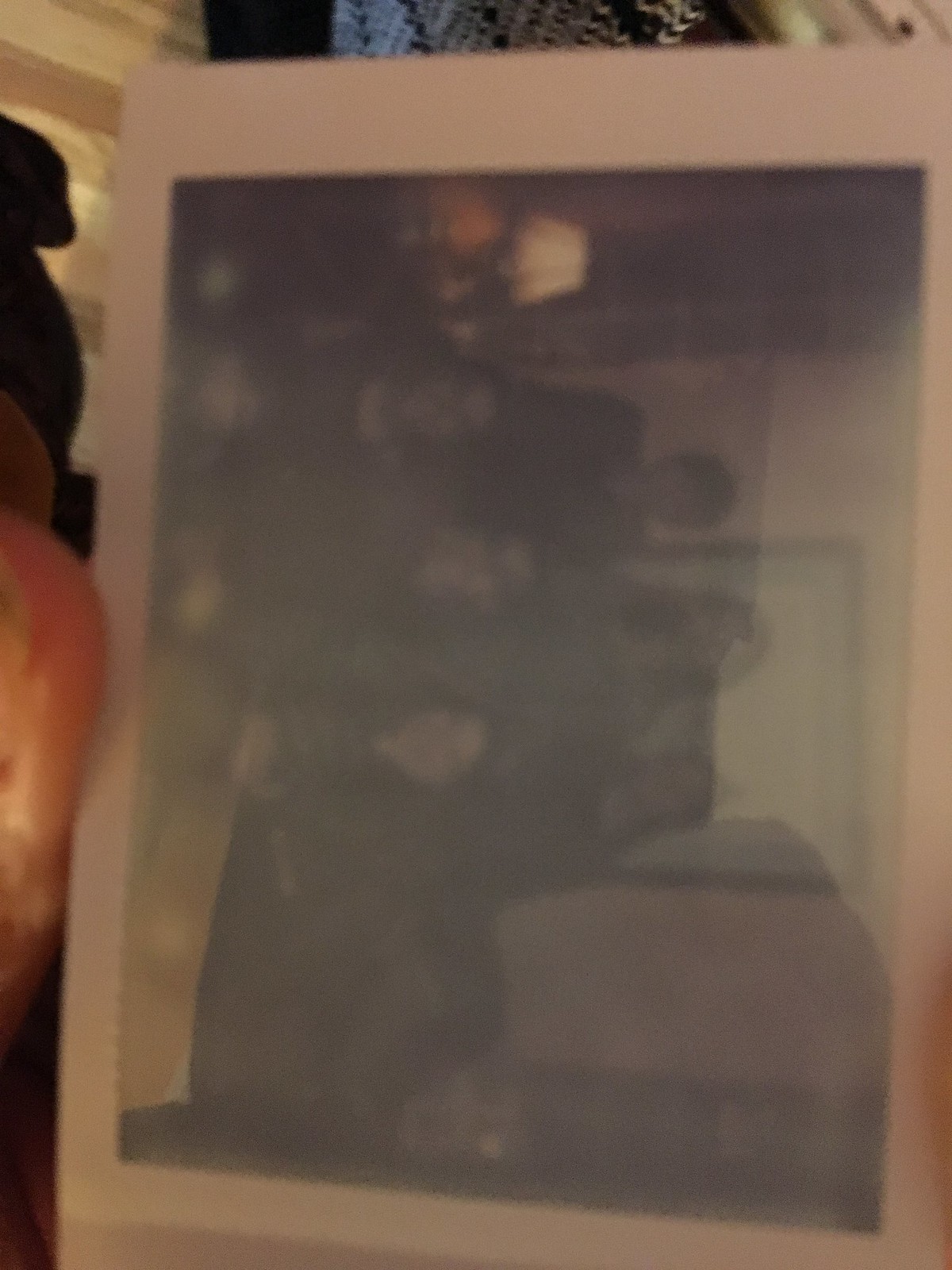In this image, a person's thumb is visible as they hold up an old, faded black and white photo. The photo itself, slightly rotated with its top on the right side, features six individuals arranged in two rows—three at the top and three at the bottom. The setting appears to be a living room; there's a small table with a lamp on it positioned to the left side of the photo. Despite the significant fading which obscures many details, the family-like grouping of the six people is discernible. The nostalgic aura of the picture hints at its sentimental value, though the wear and tear have unfortunately diminished its visual clarity.